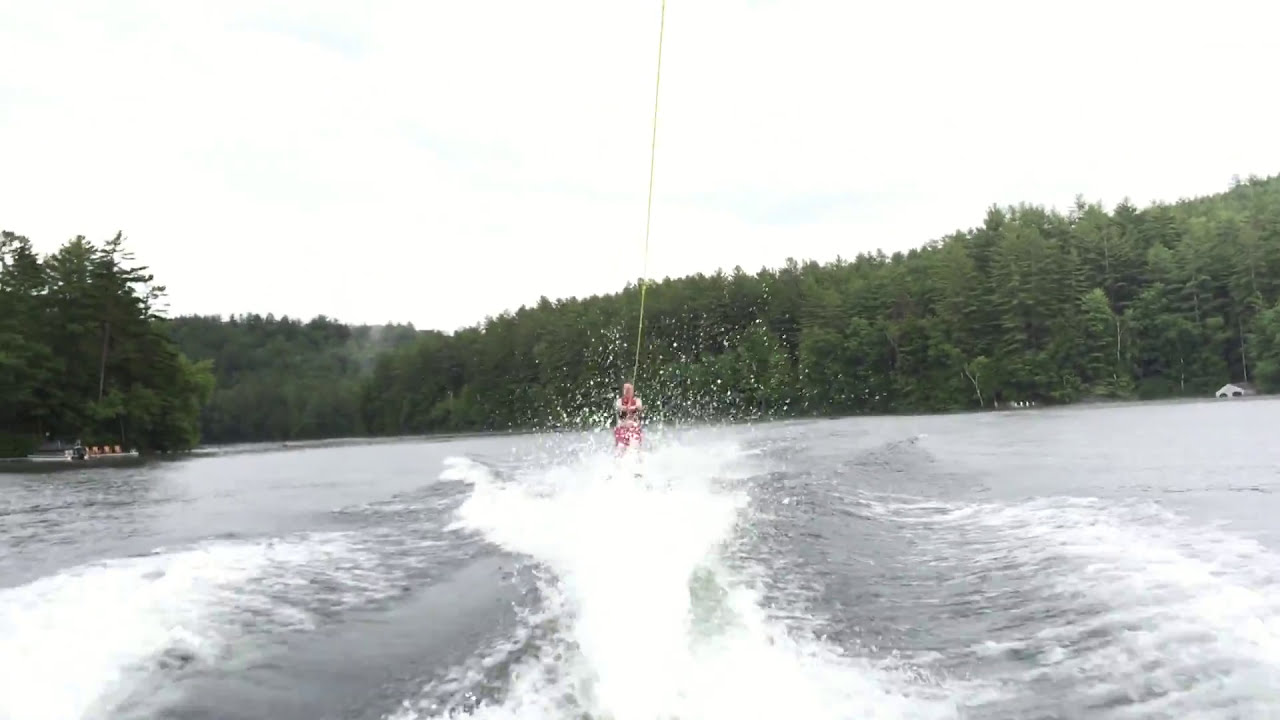The photograph captures an action-filled scene of a person waterskiing on a dark, blackish-gray lake. The skier, positioned at the center of the image, is gripping a yellow tow rope that extends down from the bottom of the image, suggesting it is attached to a boat outside the frame. The skier is adorned in what appears to be a white outfit with a red safety jacket and possibly a red helmet, though some details are inconsistent in the various descriptions. The skier glides across the water amidst frothy wake waves and white bubbles churned up by the boat's engine and their motion. Surrounding the lake are hills densely covered with green trees, likely pines. The sky overhead is an overcast, cloudy white, adding a muted tone to the landscape. The lake itself curves slightly from left to right, enhancing the sense of a dynamic, adventurous outdoor setting.